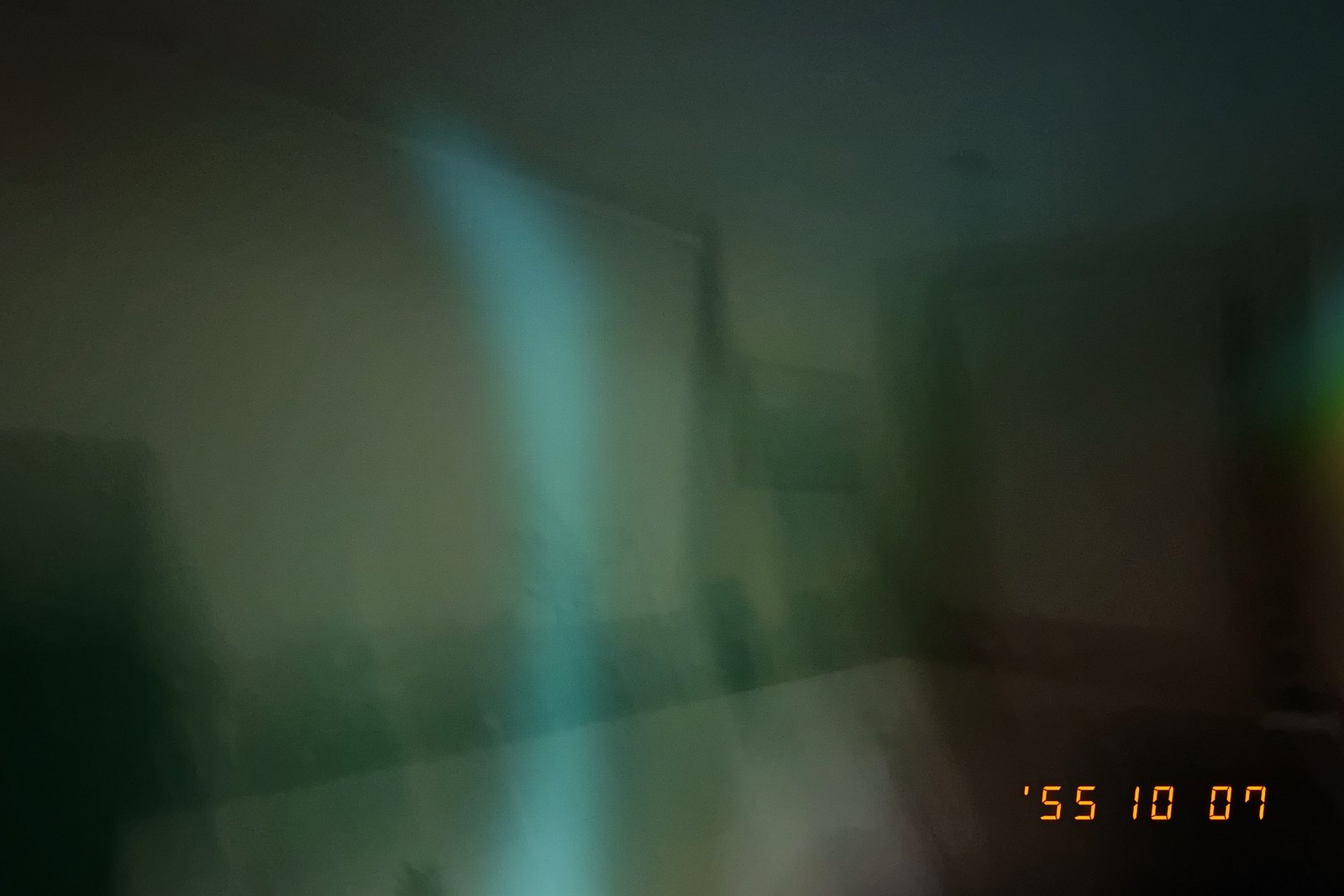This is a highly blurry and dark photograph with a discernible orange digital date stamp in the bottom corner, reading "55 10 07." The overall scene appears to be taken inside a dimly-lit room with no lights on, casting a greenish tint over the image. The room features a prominent white surface, possibly a floor or tabletop, which stretches or expands toward the edges. The top left area of the image contains a white rectangle that might represent a wall or another object, though its exact nature is unclear. The lower left corner is notably black, hinting at an object or shadow within the room. Additionally, there is a possible dark shadow or the silhouette of a TV toward the right side of the photo, with what may be a dark picture mounted on a white wall in the background. Despite the lack of clarity, the photo's composition gives an impression of looking through a window into a shadowy, indistinct space.